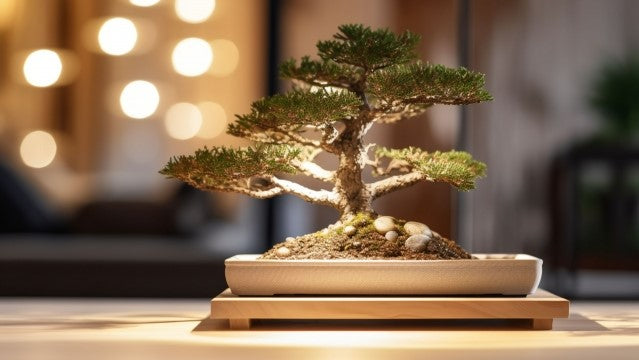This professional landscape photograph captures a close-up of a meticulously crafted bonsai tree, approximately six to seven inches tall, resembling a miniature version of a grand, iconic African yew tree. The bonsai, with its thick trunk and upward-pointing, pine-needle-like leaves, is planted in a mound of dirt adorned with a few rocks. It sits elegantly in a white ceramic tray atop a small wooden stand, which is placed on a bamboo table. The background features a softly blurred living room scene, with a blue couch on the left side and golden, fairy-like lights from windows that evoke a festive ambiance. The soft-focus effect enhances the delicate yet intricate details of the bonsai, making it the central highlight of this serene indoor setting.